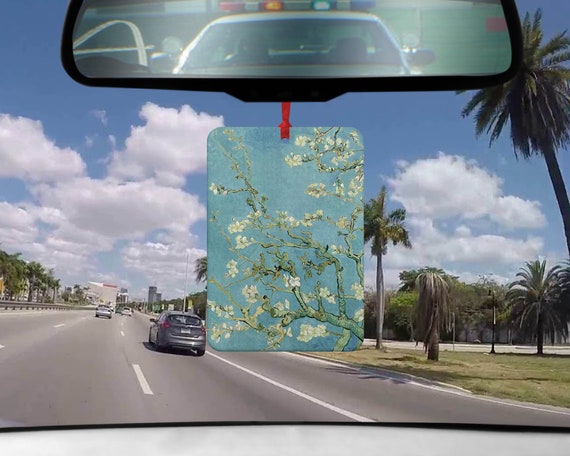This image is taken from inside a car, looking out through the front windshield onto a highway that seems to pass through a warm, possibly tropical area, likely California or Florida. The sky outside is a vivid blue with a few white clouds scattered across it. Palm trees line both sides of the road, and tall skyscraper buildings can be seen in the distance, indicating an urban setting. The road itself is divided by white lines, with several cars driving ahead.

The car's rearview mirror is prominently featured in the image, reflecting a police car directly behind. The police car has an older model look and seems to be quite close, but its lights are not flashing. Hanging from the rearview mirror inside the car is a rectangular air freshener with a floral design. The freshener, adorned with white flowers that have yellow centers and green leaves, hangs from a red ribbon and adds a touch of colorful decoration to the scene. This detailed view of the air freshener and the reflection of the police car captures the viewer’s attention, making it a key element of the photo.